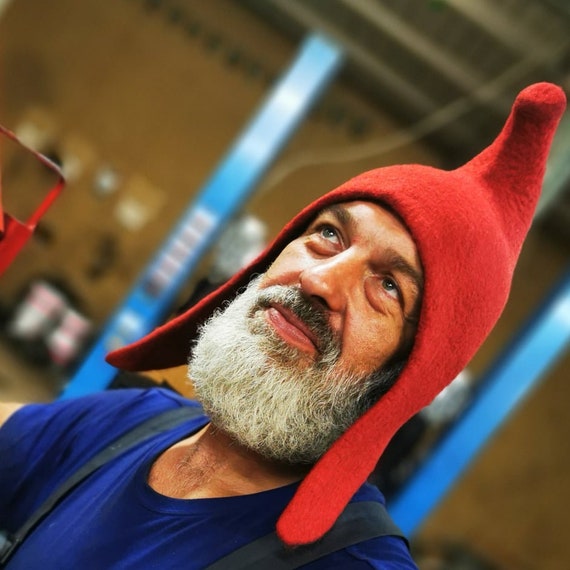In this image, a man, who appears to be around 60 years old, is depicted looking upwards and off to the right with a somewhat contented expression. He sports a big, bushy gray beard and mustache, and his green eyes are visible beneath a quirky, red felt hat. The peculiar hat features flaps that extend down to his shoulders and a pointed horn-like top, adding an intriguing, possibly festive or theatrical touch to his appearance. He is dressed in a navy blue T-shirt, which is paired with something resembling black overalls or possibly suspenders. The photograph is taken from a low, left-angled perspective that captures the man from the bottom left to the top right of the frame, enhancing the dynamic feel of the shot. The background is blurry, making it difficult to decipher the exact environment, but it hints at an industrial or workspace setting with two blue columns or support beams, a brownish wall, and some metallic elements. There is also a box nearby, contributing to the impression that he might be at his job in a mechanic's garage or similar workplace.